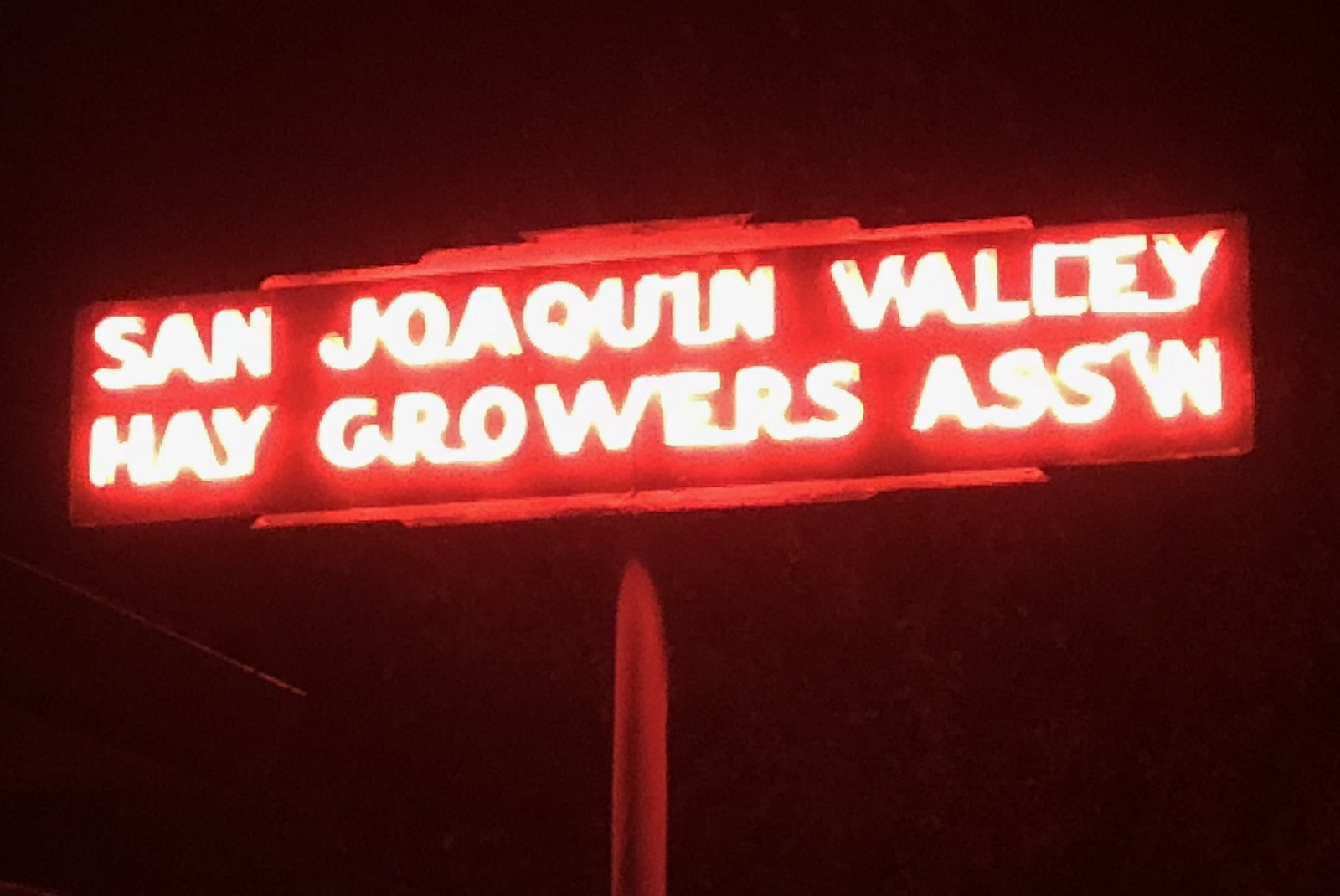This nighttime photograph features a prominently illuminated red neon billboard against a completely dark background. The billboard, overexposed due to a likely camera setting mishap, reads "San Joaquin Valley Hay Growers A.S.S.'N" with vivid, glowing letters. The bright red neon light not only highlights the bold white text but casts a strong red glow on the entire scene, including the central red pole supporting the sign. To the bottom left of the image, a faintly visible corner of a building or another structure adds a subtle contextual element. A white light streak is noticeable to the left beneath the sign, potentially indicating another light source or a reflection. The overall composition suggests this may be an outdoor advertisement, perhaps for a hotel or local establishment in the San Joaquin Valley.